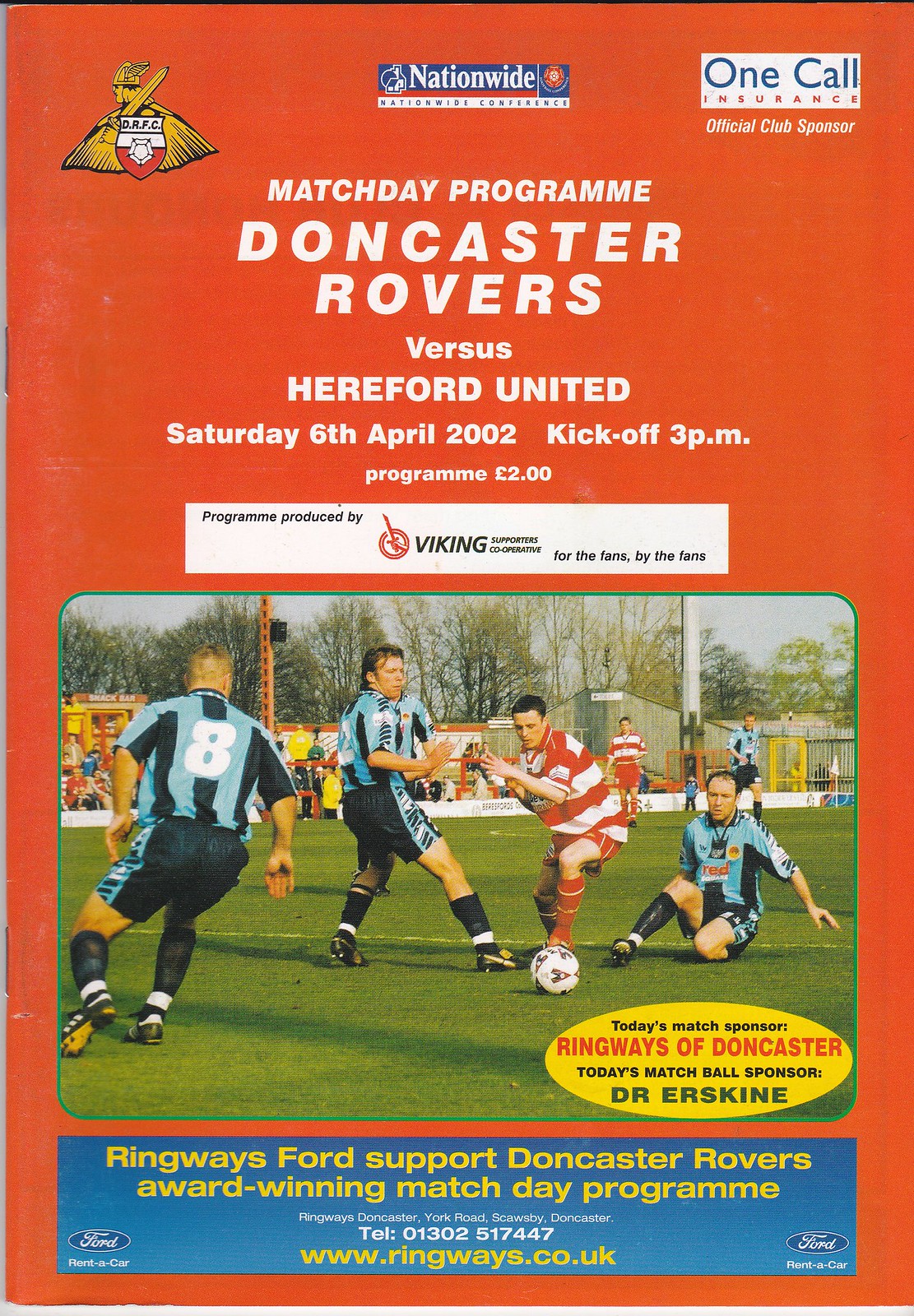The image depicts the cover of a match day program for a soccer game, set against a vibrant red background. At the top, several sponsors are mentioned, including Nationwide and One Call Insurance, alongside the official club sponsor label. Dominating the upper section is the Doncaster Rovers club logo, showcasing a viking holding a shield and sword. In prominent white text, it reads: "Match Day Program, Doncaster Rovers vs. Hereford United, Saturday, 6 April 2002, Kickoff: 3 p.m." The program is noted to be priced at two British pounds and is produced by the Viking Supporters Cooperative, emphasizing its nature "for the fans, by the fans."

The centerpiece of the cover features an action shot of a soccer match, likely an older photograph. The players are engaged in the game on a grassy field, with one team in black and blue striped uniforms, and the other in red and white stripes. In the bottom right corner, an orange circle highlights today's match sponsor, Ringways of Doncaster, and today's match ball sponsor, Dr. Erskine. Along the bottom edge, there's an advertisement for Ridgway Ford, stating their support for the award-winning match day program. This detail underscores the local car dealership's involvement in sponsoring the publication.